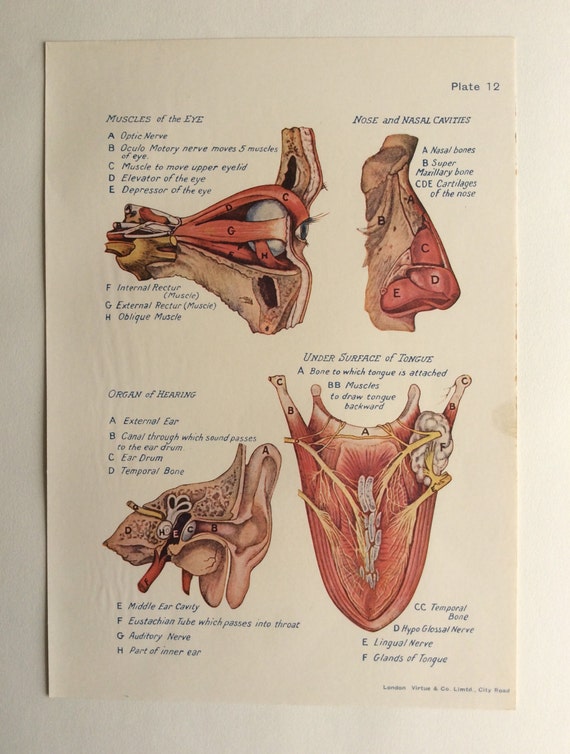This image is a detailed, vintage medical anatomy illustration labeled "Plate 12," originating from a textbook. It features cross-sectional diagrams of various facial anatomical structures including the eye, nose, ear, and tongue. 

At the top left, the section labeled "Muscles of the Eye" is annotated with letters pointing out the optic nerve, oculomotor nerve responsible for moving five eye muscles, the muscle controlling the upper eyelid, and the muscles that elevate, depress, and move the eye laterally (internal and external rectus muscles) as well as the oblique muscle.

To the right, the illustration of the "Nose and Nasal Cavities" identifies the nasal bones, the supramaxillary bone, and various cartilages forming the nose structure.

Below and to the left, the section titled "Organ of Hearing" displays the external ear, the canal leading to the eardrum, the eardrum itself, the temporal bone, the middle ear cavity, the Eustachian tube connecting to the throat, the auditory nerve, and parts of the inner ear.

At the bottom right, the diagram labeled "Under Surface of Tongue" points to the bone to which the tongue is attached, muscles that retract the tongue, the temporal bone, the hypoglossal and lingual nerves, and the glands of the tongue.

Each section is meticulously labeled with letters corresponding to specific anatomical features, and blue headings organize these features into easily identifiable categories for educational purposes. The page also contains some copyright information at the bottom that is unclear.